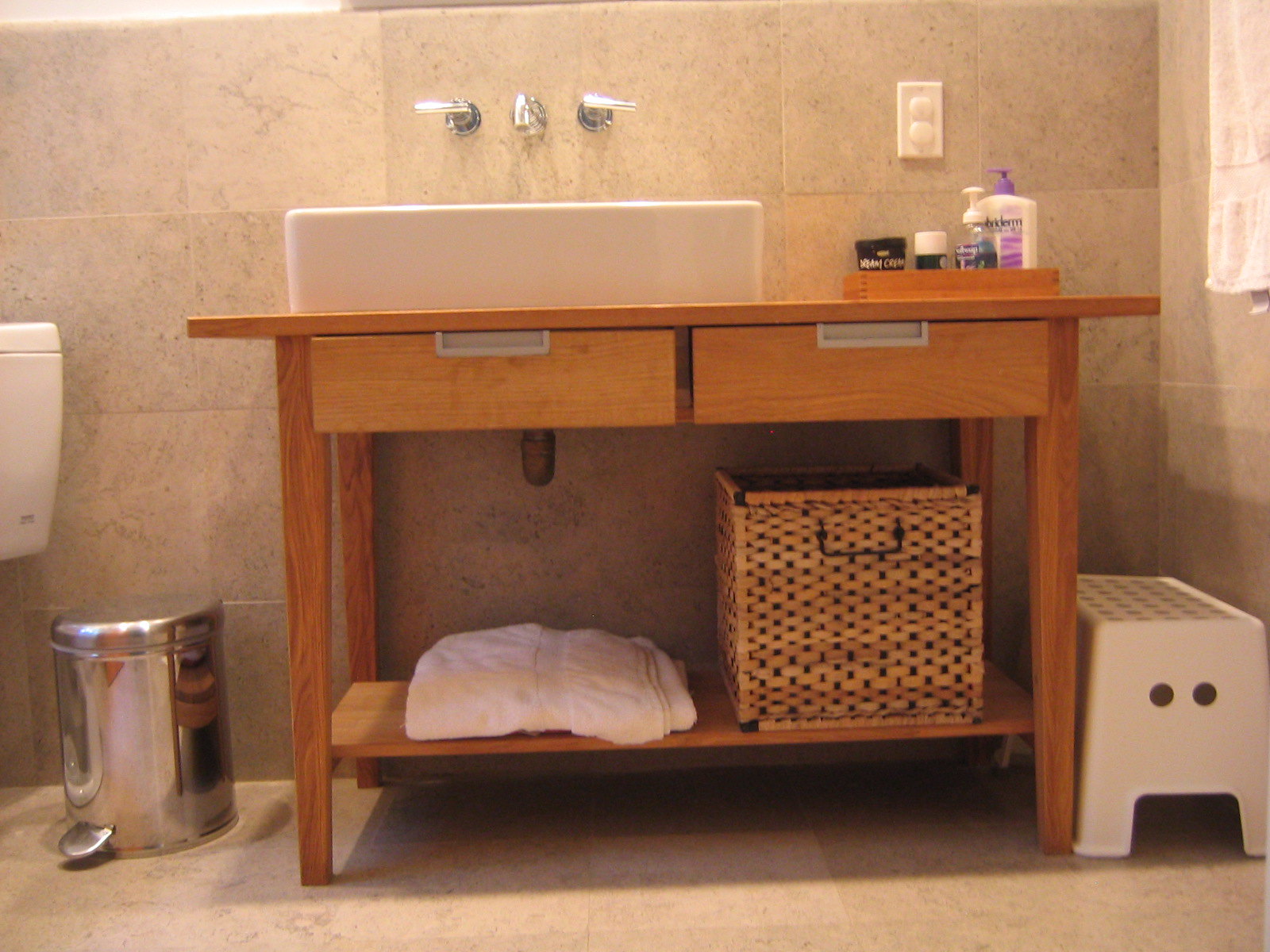In this image, a pristine white sink base is prominently displayed on a wooden table. The wall-mounted sink features a gleaming surface, contributing to the clean and orderly aesthetic of the space. Located at the back right of the sink, a white electrical plug with a plastic cover is visible, providing a subtle yet necessary detail. 

Below the table, there is a brown wicker basket, adding a touch of warmth and texture to the otherwise monochromatic color scheme. Adjacent to this, a white stool is positioned to the bottom right, complemented by a neatly folded white towel resting nearby on the pristine white floor.

To the bottom left, a compact trash can is placed efficiently beside the toilet, which is seen to the left side of the frame, showcasing just the bowl of the toilet. 

On the right side of the wooden table, various creams, lotions, and toiletries are neatly arranged in a small wooden basket, contributing to the organization and functionality of the space. Overall, the composition of the image is thoughtfully curated, emphasizing both utility and aesthetics.